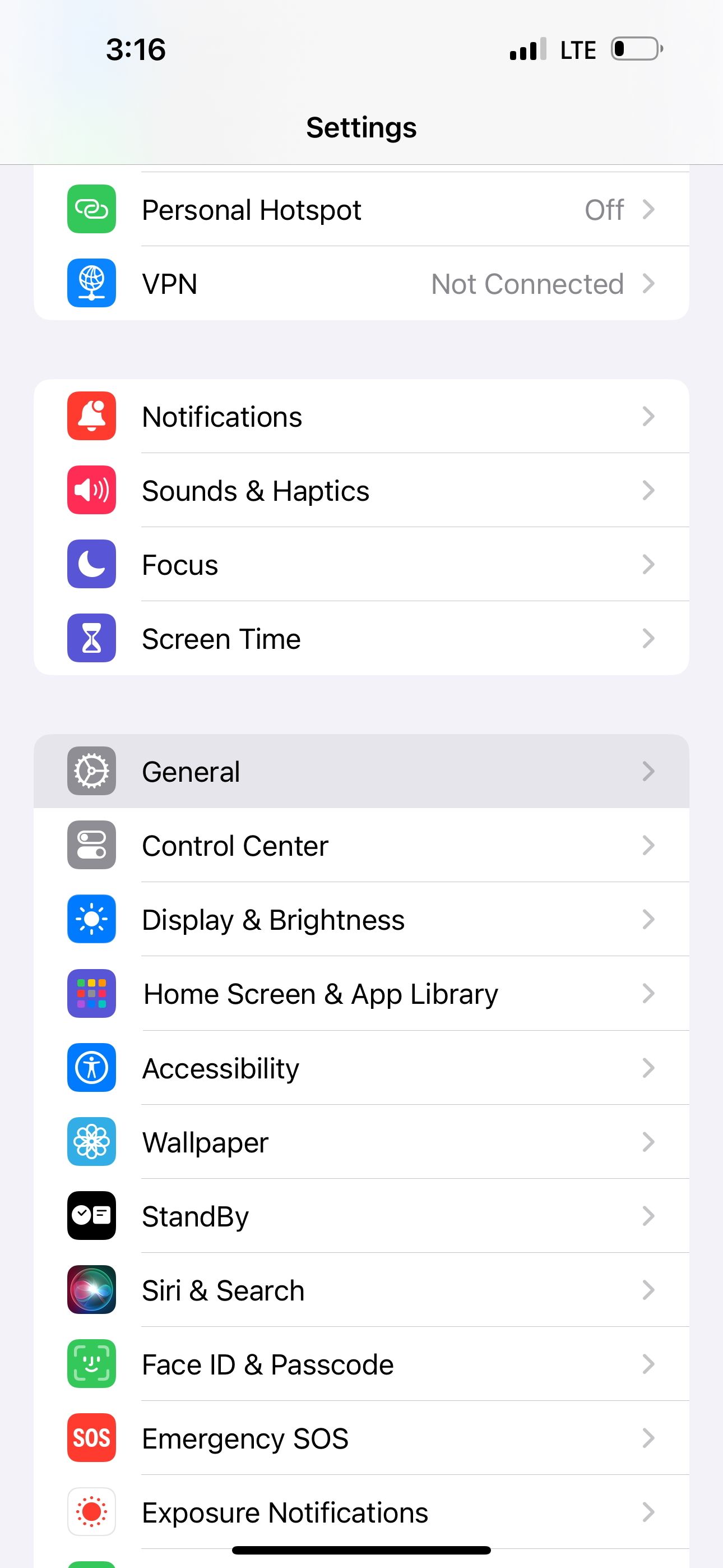The screenshot captures the settings app on an iPhone. In the upper left corner, the time is displayed, while the upper right corner features indicators for signal strength (five vertical bars; the first three are black and the fourth is gray), LTE connectivity, and a low battery icon. Below the header, the image shows several settings menu options including: Personal Hotspot (status: off), VPN (status: not connected), Notifications, Sound & Haptics, Focus, Screen Time, General (highlighted), Control Center, Display & Brightness, Home Screen & App Library, Accessibility, Wallpaper, Standby, Siri & Search, Face ID & Passcode, Emergency SOS, and Exposure Notifications.